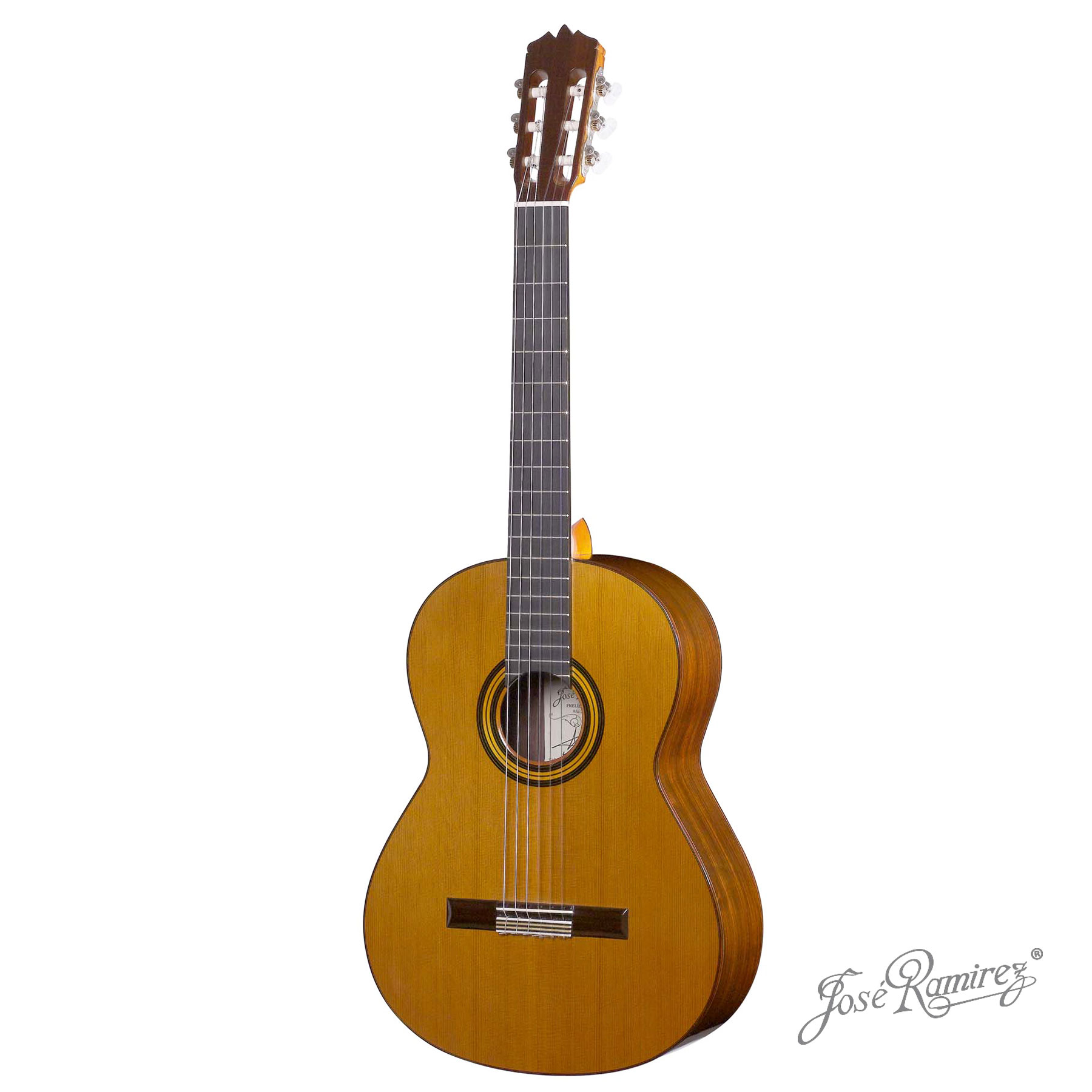The image displays an acoustic guitar positioned upright on a pure white background. The guitar has a figure-eight body shape with the front panels crafted from pale yellowish wood, while the sides and the rounded body feature slightly darker tones. In the center of the guitar's body, there is a sound hole encircled by concentric decorative bands in varying shades of brown and yellow. The fretboard and neck, made of darker wood, contrast the lighter body and display horizontal silver lines. The neck culminates in a headstock characterized by a dark wood with white accents and cut-out designs on both sides. Six metal strings run from the body to the headstock, where they are anchored by six pegs. In the bottom right corner of the image, the brand name "Jose Ramirez" is written in italic cursive, followed by an ® symbol indicating a registered trademark. This signature also appears inside the guitar, visible through the sound hole.